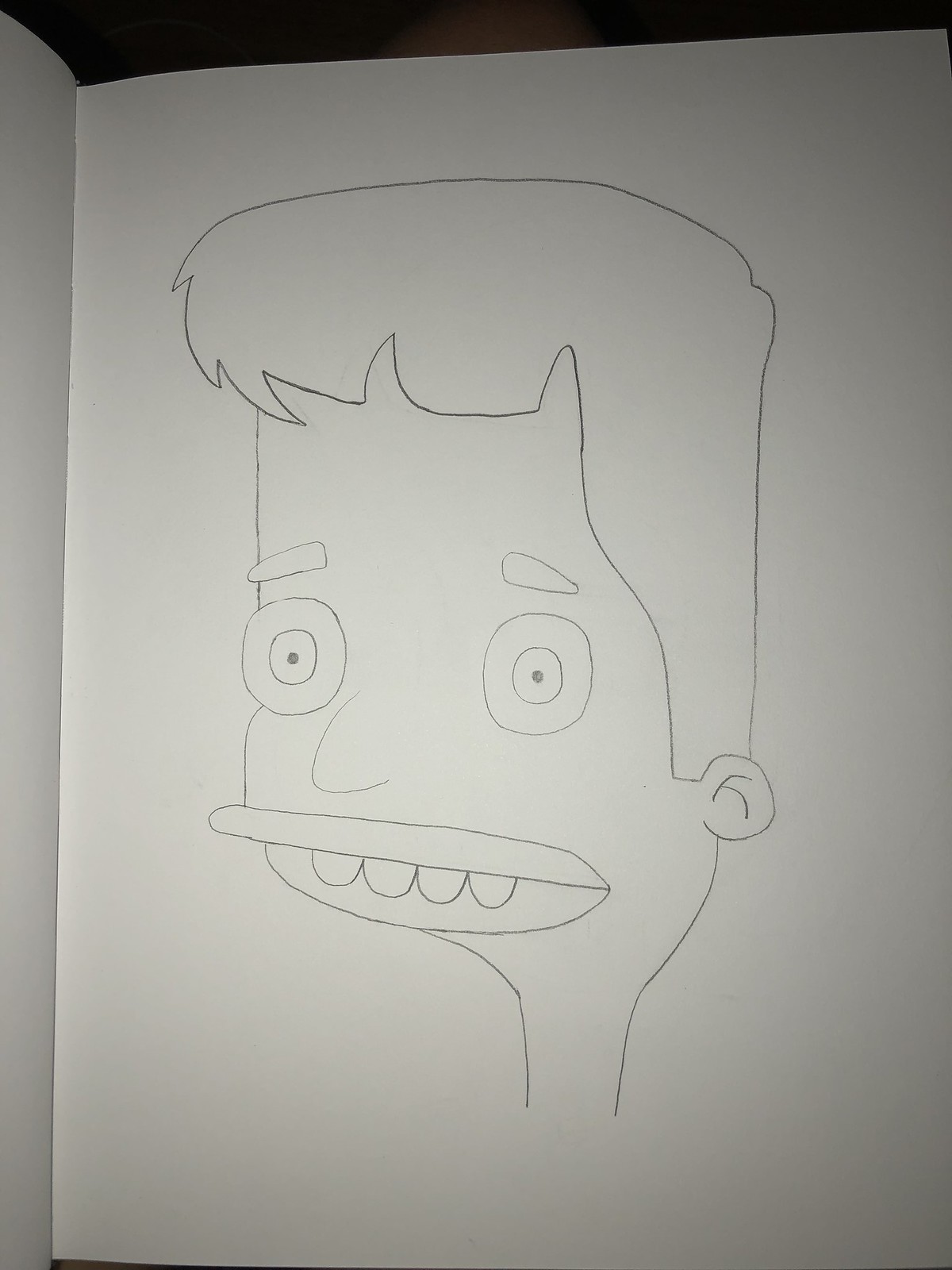This is a black-and-white photograph of a simple, cartoon-like drawing of a boy. The drawing is done on an A4-sized white sheet of paper, possibly within a booklet. The boy depicted has exaggerated facial features, including large, round eyes with concentric circles that impart a surprised expression. His eyebrows are small and positioned close to his eyes, which are in turn close to his mouth, leaving his large forehead prominently exposed. The mouth is drawn with four protruding upper teeth that are visible even though the mouth is closed. His hair is short and extends to about ear-length, framing his small ears. The neck is unusually long and slender, and the drawing halts at the neck, adding to the stylized, disproportionate appearance of the character. The overall impression is reminiscent of a crude, hand-drawn cartoon, somewhat akin to the style seen in "The Simpsons" but less detailed.